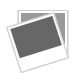The image depicts an antique decorative object centered against a textured beige background with darker shading. The object features a circular, ring-shaped base adorned with intricate gold designs. Nothing is placed within this circular slot. Extending from the base is a curved, gold-decorated stem that supports an old-looking, round brown container. This container, which resembles a cup or bowl, appears mostly empty except for the tip of something white visible inside. The entire piece exudes an outdated and possibly antique aesthetic, enhanced by the background's aged and stained appearance.